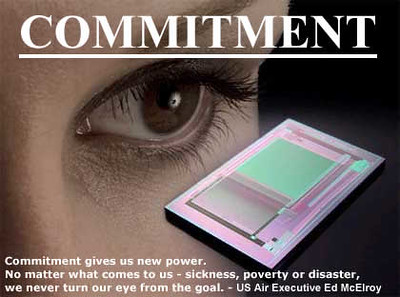In this striking close-up photograph, a woman's left eye is prominently featured against a black background. Her eye is dark brown with thick, mascara-coated lashes and makeup, including eyeliner and eyeshadow, meticulously applied. Her light skin contrasts with the dark, detailed features of her eye, capturing every granular detail of her lashes and the curve of her upper nose. The upper part of the image displays the word "COMMITMENT" in white, bold, capitalized block letters, underlined for emphasis. Beneath, a motivational quote in smaller white script reads: "Commitment gives us new power. No matter what comes to us, sickness, poverty, or disaster, we never turn our eye from the goal." The quote is attributed to U.S. Air Executive Ed McElroy. Besides her eye, on the lower right corner, there is a rectangular makeup palette with a black bottom and an effervescent pink border. It contains two compartments: one empty and the other filled with a mint green eyeshadow, reinforcing the advertisement-like feel of the image.